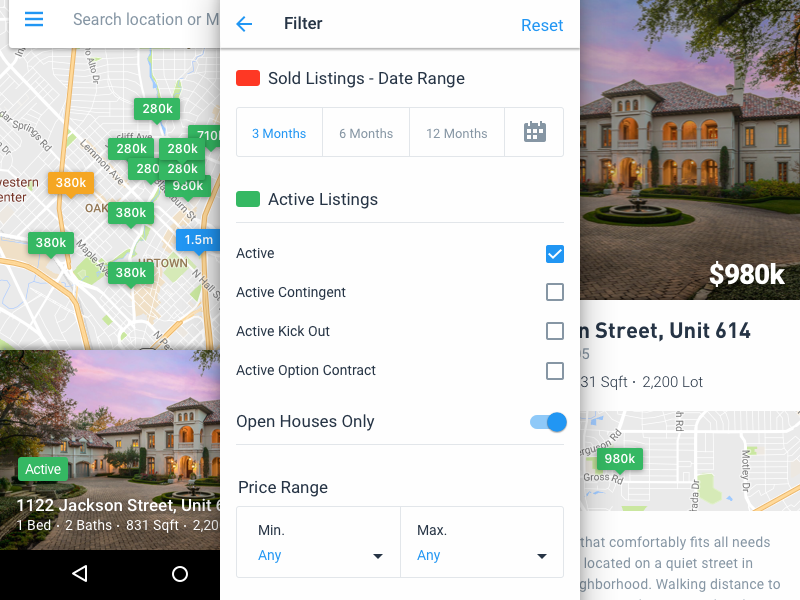The image features a white background divided into three main sections. 

On the left is a small white search box containing three blue lines and the text "Search location." 

The central portion displays a detailed map adorned with green, yellow, and blue markers. Beneath the map is an image of a large, beautiful house located at 1122 Jackson Street, described as having one bedroom and two bathrooms. This section also includes a green button labeled "Active." The bottom part of this section features a black background with a left arrow inside a circle, followed by a dropdown menu labeled "Filter." This dropdown menu, also white, includes options like "Reset," a line separator, a red box for "Sold Listings," and parameters for "Date Range" with "Three months" highlighted. 

On the right, there is a section for active listings marked by a small green box with the word "Active" and a blue box with a check mark. There's also an "Open Houses Only" option with a blue sliding toggle. Below, there are fields to input a price range with "Minimum" and "Maximum" set to "Any." 

Finally, on the far right side, there is a prominent image of a stunning house priced at $980,000. Below this image is a small map with a green marker indicating the address, followed by some blue text.